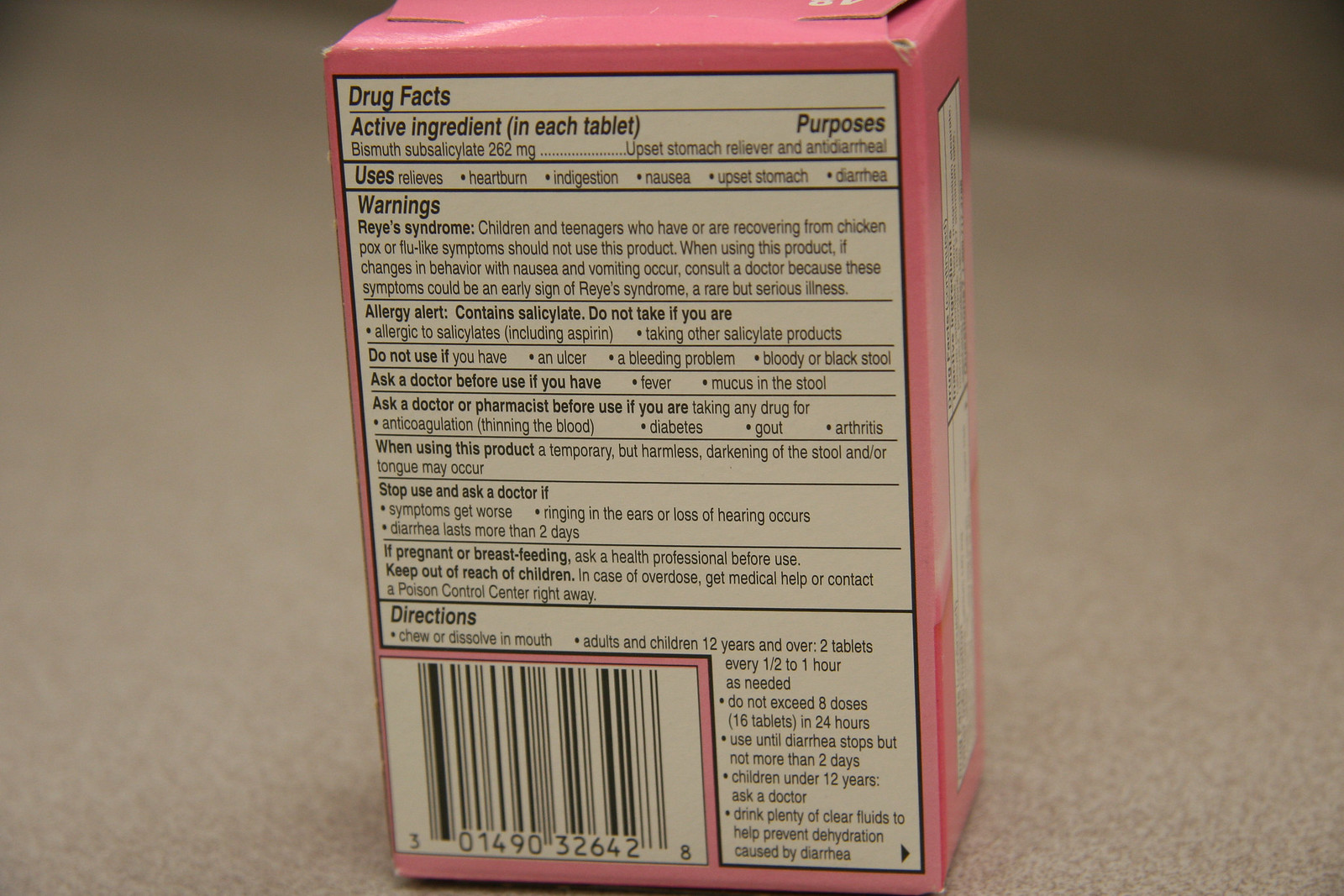In this highly detailed photograph, we observe the back of a Pepto-Bismol box, displaying extensive pharmaceutical information. The box is vividly colored in a light or hot pink hue, enhancing its visibility. Prominent on the back of the box are the "Drug Facts," starting with the "Active Ingredient" section. The product’s key uses are clearly listed, providing relief for heartburn, indigestion, nausea, upset stomach, and diarrhea. 

The image also conveys critical safety information, including warnings about Reye's syndrome and an allergy alert emphasizing that the product contains salicylate. It advises individuals not to take Pepto-Bismol if they are allergic to salicylates or are using other products that contain it. 

Furthermore, there is an advisory to consult a doctor before use, with a specific mention to review a listed set of conditions. Instructions recommend discontinuing use if symptoms worsen, if there is ringing in the ears, or if diarrhea persists for more than two days. This detailed information is pivotal for ensuring the safe and effective use of the medication.